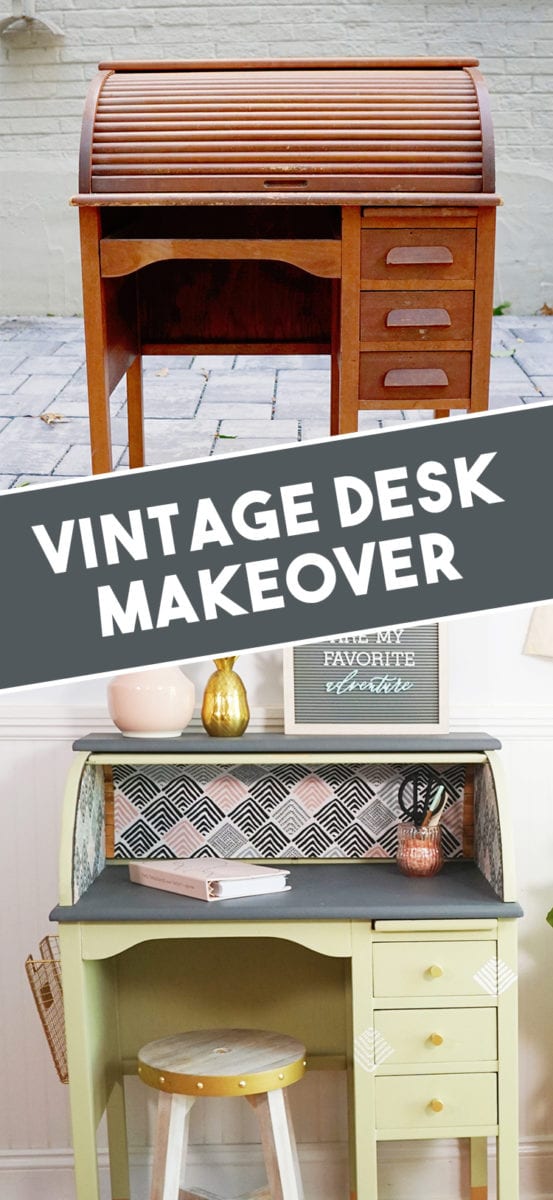The image shows a compelling before-and-after transformation of a vintage desk, divided into two distinct sections by a dark gray banner with white text reading "Vintage Desk Makeover." In the 'before' section, the desk is positioned on a cement walkway with a white brick wall in the background. The desk, made of darker wood, features an accordion-style flip-up top and appears worn and aged.

The 'after' section reveals the revitalized desk, presenting significant improvements and a modern aesthetic. Painted in a light yellow hue, the desk now boasts smaller, matching yellow knobs, and its interior has been adorned with a dynamic black, gray, and pink wallpaper-like material. A new gray countertop has been added, enhancing its functionality and appearance. The desk is open, showcasing the creative makeover. Accessories like a pink book, a peach vase, and a golden transparent vase sit atop, adding charm. The transformation is complete with a stool placed underneath and a framed print on the left side reading “my favorite.” The desk now resides in a home setting, providing a stark contrast to its previous condition.